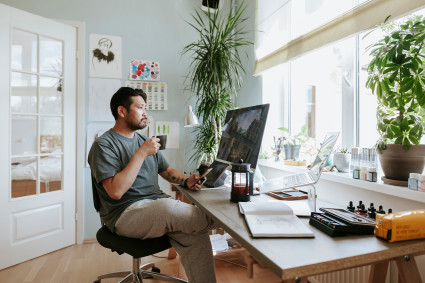In this detailed photograph of a home office, a man with brown hair and a beard, who appears to be of Indian or Asian descent, is seated at a thin desk, engrossed in a monitor. He is wearing a greenish-colored shirt and khaki pants, with his right leg crossed over his left, holding a coffee cup in his right hand and a cell phone in his left. Surrounding him, the room features various elements including a large grey wall adorned with hand-drawn pictures and posters positioned prominently in the center of the background. To the left of this wall is a white door inset with glass windows, and to its right are expansive glass windows, potentially shaded, through which one can see outside. The scene is punctuated by greenery: a tall plant stretches upward toward the ceiling from a corner, and another plant in a ceramic pot occupies the window on the right side of the image. Additional shelves, lined with various knick-knacks and ceramics, hold more plants. Elements typical of a work environment, such as a book or manual and possibly a calculator, are present on the desk, indicating that the man is likely engaged in morning work tasks.